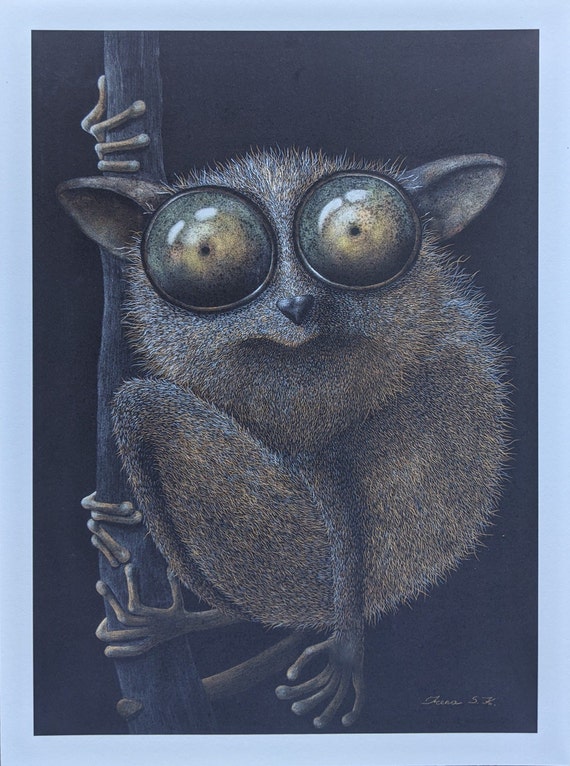The image showcases a detailed drawing of a small, primate-like creature with a compact, circular body covered in spiky, brownish-gray fur. The animal, which is clasping a small tree branch with both its hind feet and right hand while its left hand dangles by its side, has strikingly large, button-like eyes that appear glassy and prominently occupy half of its face. These eyes are notable for their teal color with gray outer rings and light yellow centers, giving it a surprised and endearing expression. The creature's pointy ears, situated on either side of its head, add to its expressive features. The dark, almost black background contrasts sharply with the creature's fur, and the artwork is bordered by a thin, light blue frame. In the bottom right corner of the image, the artist's signature, possibly reading "Icena 5X," is faintly inscribed.